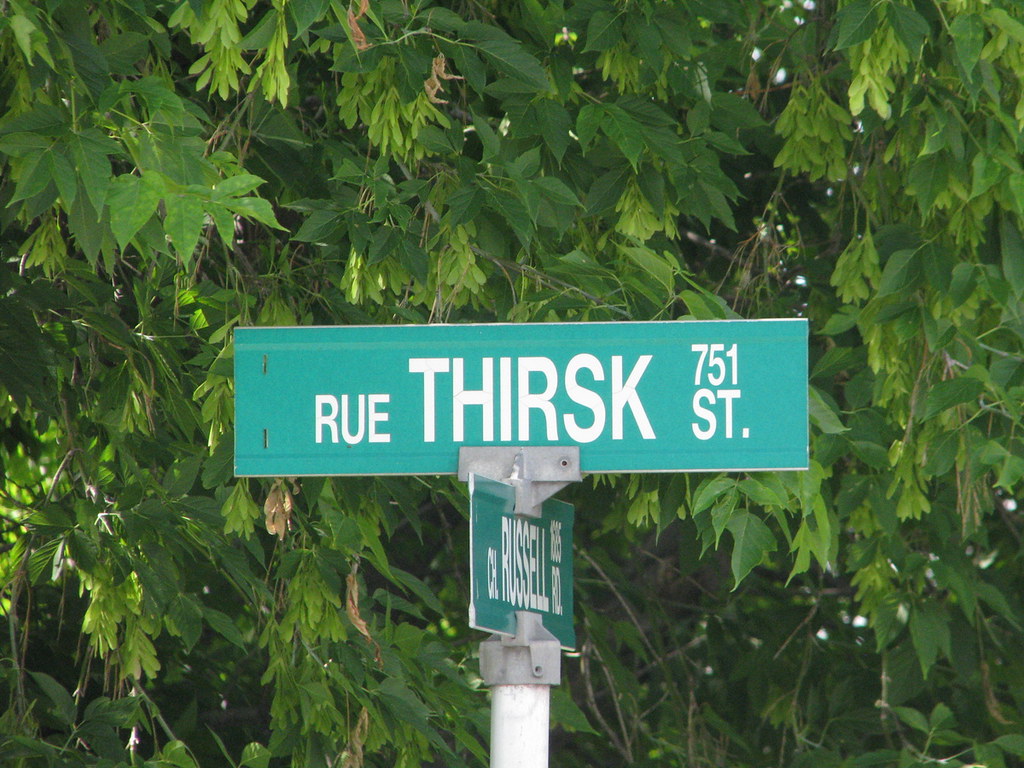This detailed photograph captures a street sign at the intersection of Rue Thirsk Street and CH Russell Road. The image is of high clarity, showcasing every detail with precision. The sign comprises two green panels with white text. The primary sign, Rue Thirsk Street, appears prominently in the foreground, displaying "751ST." The secondary sign for CH Russell Road is angled to the side, reading "1555RD." Both signs are mounted on a weathered white pole, which shows signs of discoloration and rust, connected using gray metal brackets. The backdrop features lush green foliage, with some leaves exhibiting brown hues, indicative of the changing season. This serene setting, likely located in a place like Quebec or Nova Scotia, is captured in a crisp and detailed manner.